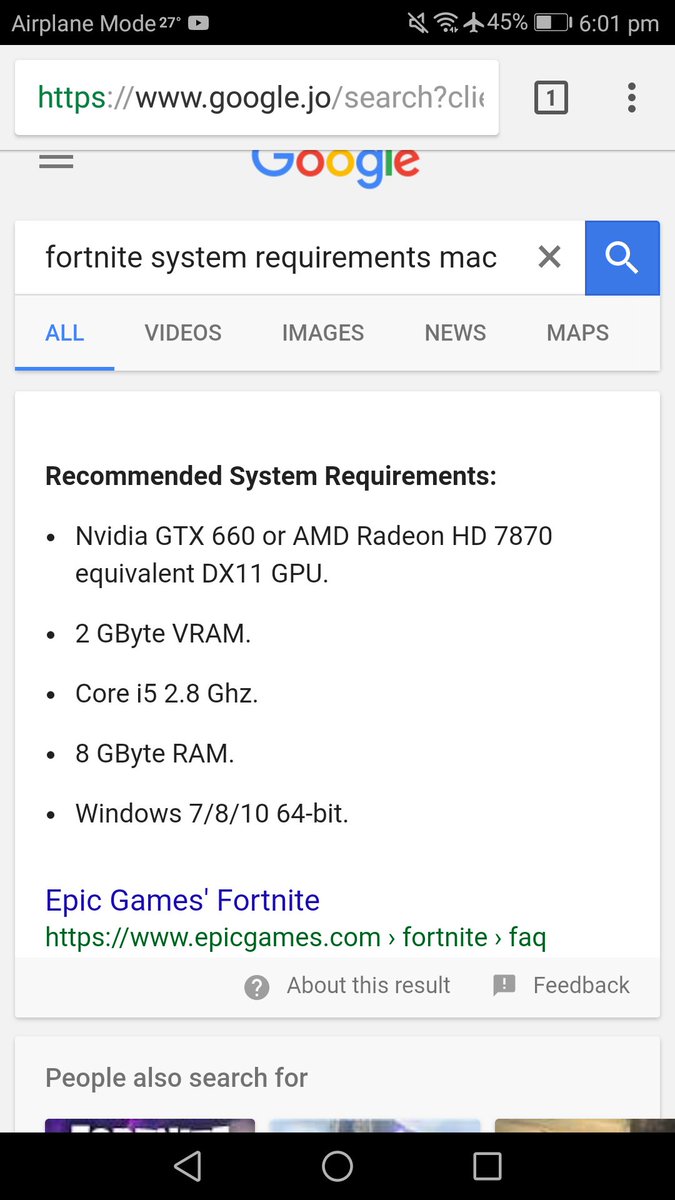**Detailed Caption:**
The image depicts a cell phone screenshot displaying search results for "Fortnite system requirements." The device is a Mac, as indicated by the presence of Mac-specific icons and layout. On the top left-hand corner, the phone is shown to be in airplane mode, with a current outside temperature of 27 degrees displayed beside it. Adjacent to the icons, a YouTube play button icon is visible. On the top right-hand side, the time is marked as 6:01 p.m., and the battery level is at 45%. Additional status icons include the airplane mode icon, Wi-Fi signal icon, and a "no ringer" icon, indicating that the phone's ringer is turned off.

Beneath these status indicators is a single open tab showing the Google web address. The search bar reflects a query for "Fortnite system requirements," revealing the recommended specifications listed below: 2 gigabytes of VRAM, a processor with a core speed of 2.8 gigahertz, and 8 gigabytes of RAM.